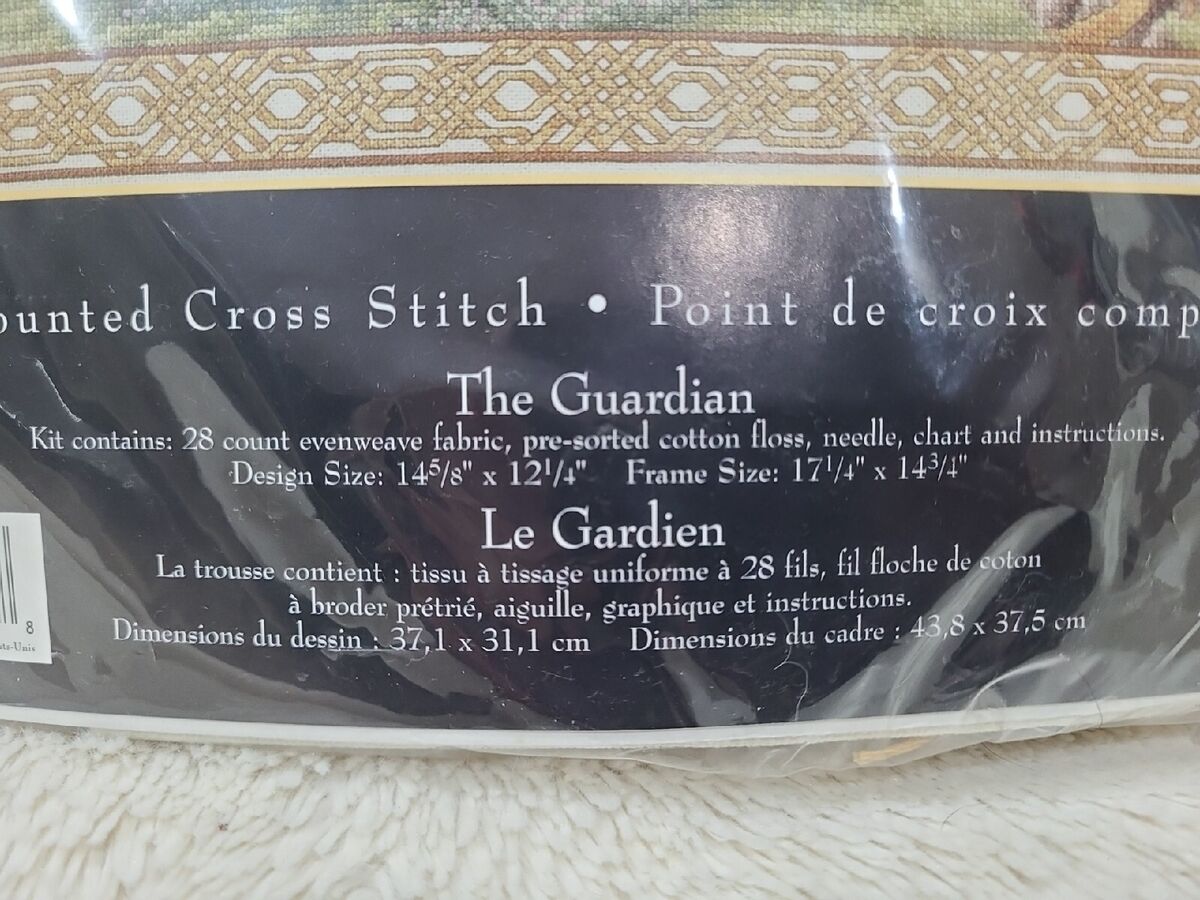This is a close-up image of a cross-stitch kit packaging encased in heavy plastic, set against a cream-colored, long-shag carpet. The black label inside the packaging features white text in both English and French. The top portion of the label shows a segment of the cross-stitch design, depicting a woven Celtic braid pattern. The text beneath the design reads "Counted Cross Stitch" and "Point de Croix," followed by an incomplete phrase. The main title of the kit is "The Guardian." The contents listed include 28-count even weave fabric, pre-sorted cotton floss, a needle, a chart, and instructions. The design size is specified as 14 and 5/8 inches by 12 and 1/4 inches, and the frame size is 17 and 1/4 inches by 14 and 3/4 inches. This information is also provided in French below the English text.